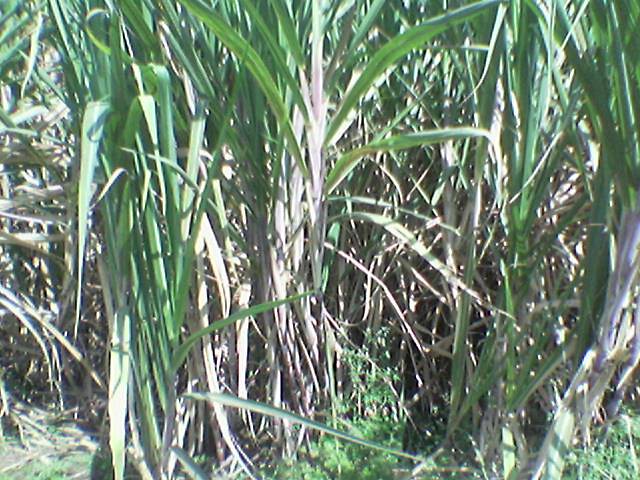This is a bright, outdoor, square image taken during the daytime, predominantly featuring tall blades of grass and weeds. The ground is visible in the lower corners, showing sparse patches of shorter grass, some brown, dead spaces, and occasional dirt. Dead branches lie atop the grass in the lower section. The majority of the image is filled with vertical strands of grass, half of which are green and the other half brown. Some of the greener blades appear to be sprouting from the brown, dead ones, with a mix of upright and sideways-turned stems. No animals, text, or other objects are present, making the focus solely on the interplay between the green and brown vegetation.